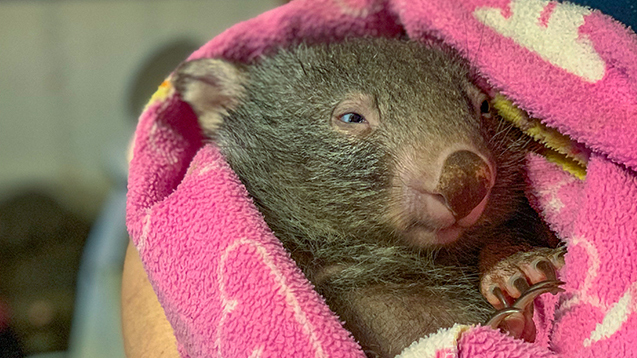The image features a close-up view of a young baby wallaby wrapped snugly in a bright pink blanket decorated with white cloud patterns. The wallaby, with its gray beige fur and prominent long claws, appears to be sleeping peacefully, facing slightly to the right. The wallaby's small beady black eyes and big brown nose contrast with patches of bare, pink skin around its eyes and nose. The delicate paws are extended outward, showcasing its lengthy nails. The background is blurred, revealing just a hint of a white wall and brown furniture, accentuating the focus on the wallaby. A light-skinned person, likely an adult, is gently holding the tiny creature, emphasizing the cuteness and tenderness of the moment.